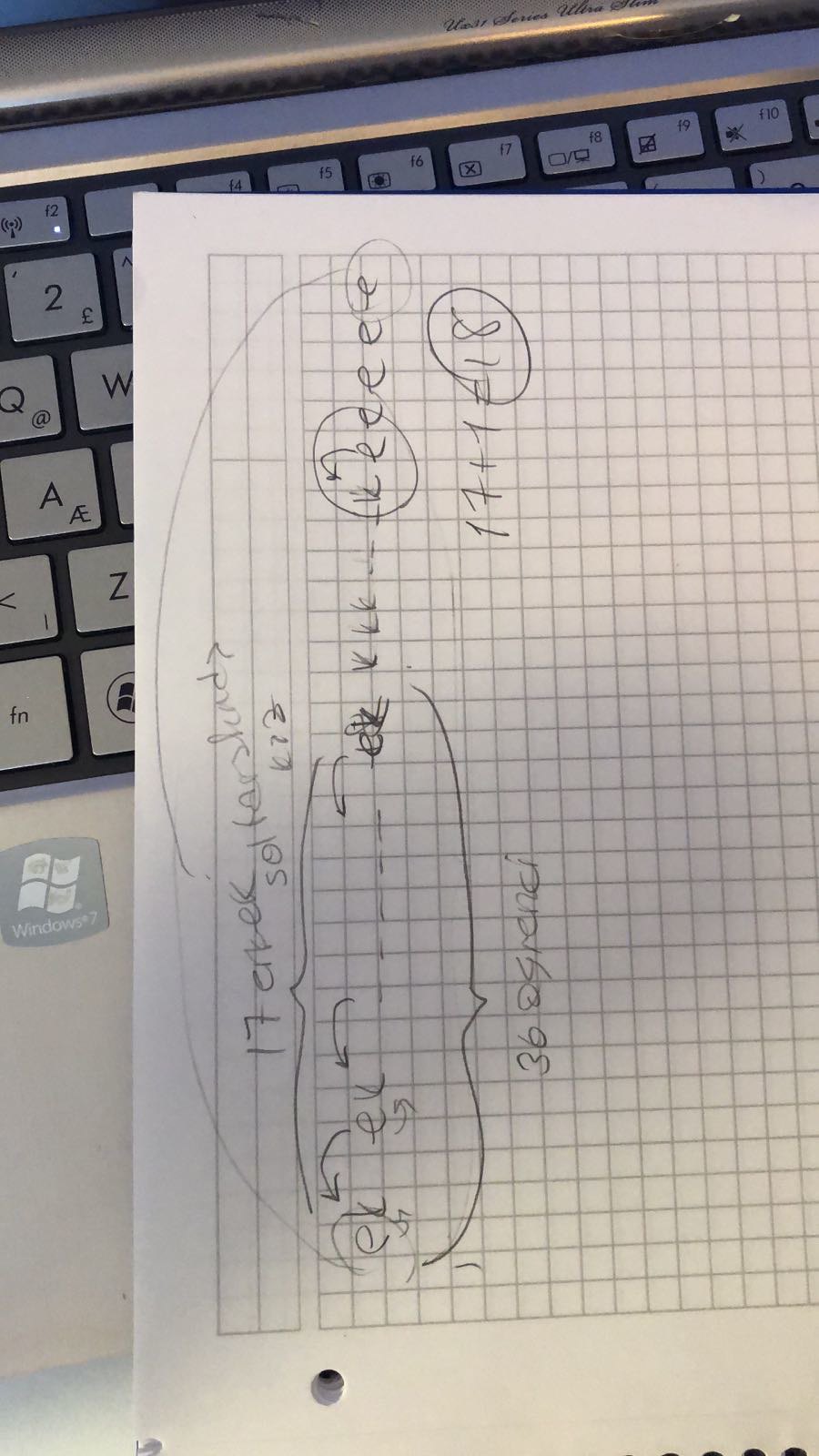The image depicts a laptop keyboard, running Windows 7, partially obscured by a graph paper notebook laid across it at an angle. The notebook contains handwritten notes, featuring various numbers and formulas. Among the legible elements, "17" can be seen, along with a formula involving "EK" followed by an arrow and another "EK." Below this, "36" is partially decipherable, along with a sequence of letters including "KKK," "K," "EE," and several E's that are circled. Another mathematical note reads "17 + 1 = 18," with the resulting "18" circled. The scene is well-lit, suggesting either strong artificial lighting or natural light streaming in from a nearby window. Additionally, the button above the "2" key on the laptop keyboard has a small dot illuminated in its bottom left corner.